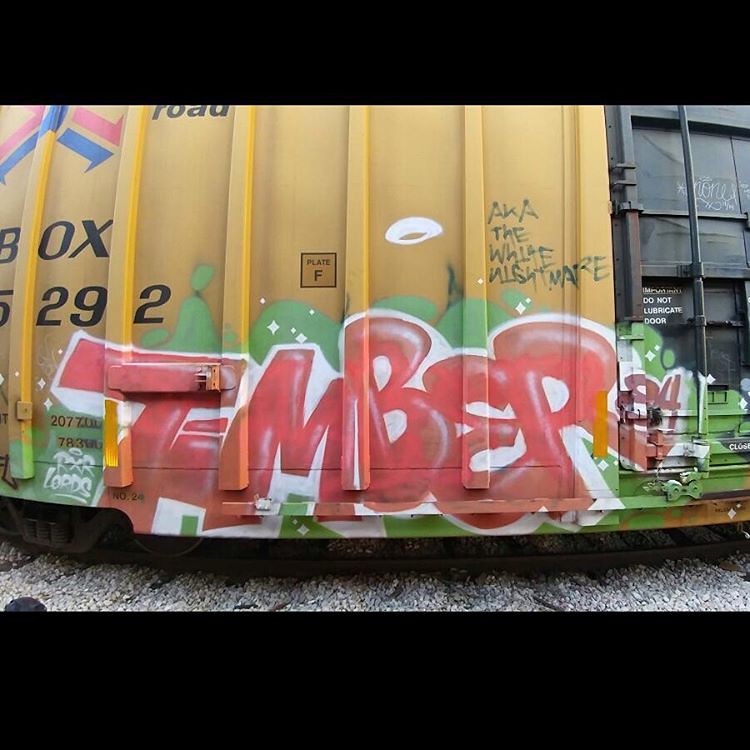This detailed photograph captures the side of a yellow boxcar decorated with vibrant graffiti. The train, identified as boxcar number 5292 and marked with "Plate F," is connected to a gray train box. The graffiti sprawls across the bottom portion of the car, showcasing the word "T-M-B-E-R 84" in prominent red bubble letters with a white border, set against a green cloud-like background. Above the "R" in the graffiti, the phrase "AKA, the White Nightmare" is visible. Additional graffiti includes "RXR Lords" with a halo above the "X." The side of the train car displays ridges resembling support beams, and large black identification numbers are present on the left side, along with a logo of a freight company featuring a red and blue symbol. In the foreground, the image captures the metal train tracks and surrounding pebbles. Notably, no people are present in this photograph, and both blue and red painted arrows are seen on the train's surface.